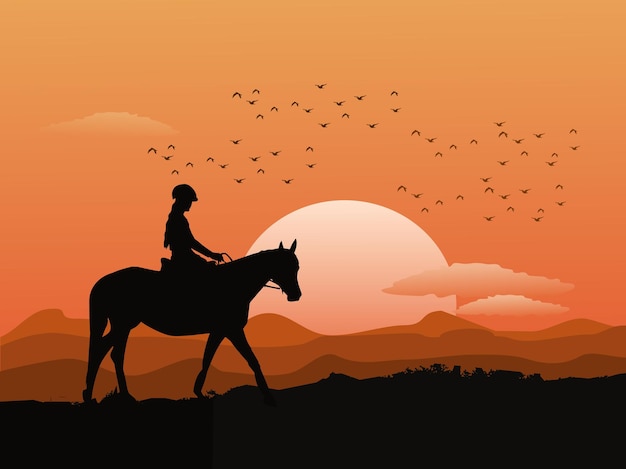This image is an abstract silhouette artwork depicting a solitary scene of a female rider with long hair and a helmet, trotting along on a horse. The silhouettes of both the rider and horse are starkly dark against a vibrant backdrop. The sky dominates the top portion of the image, painted in a light sherbet orange hue, transitioning to shades of amber and brown towards the horizon, where a pale sun is setting. In the background, we see a few clouds—one situated in the top left corner and two more in the lower right midsection. Adding to the serene ambiance, a flock of birds is depicted flying across the sky. The landscape below the horse and rider silhouettes is also dark, creating a stark contrast with the bright and warm colors of the setting sun and the surrounding hills.